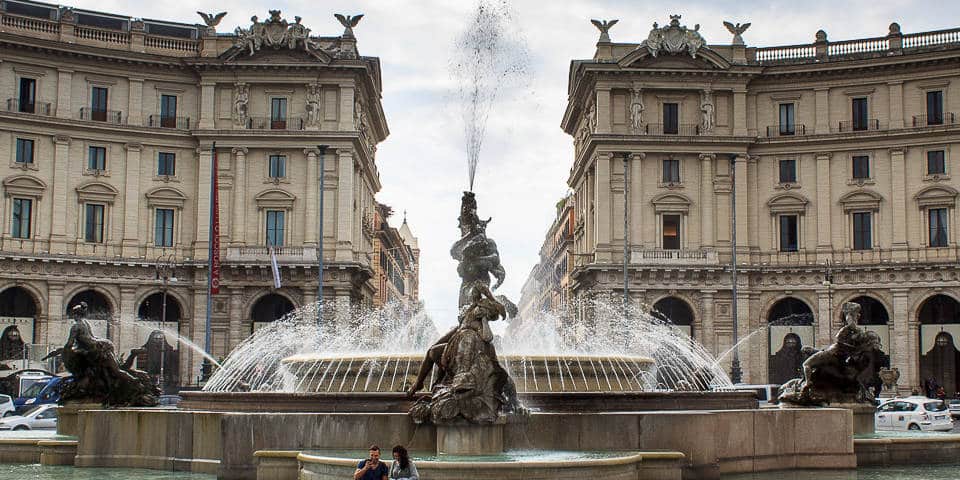The image captures a European-style city center dominated by two intricately ornate, mirror-image buildings flanking either side of the frame. These historic, possibly British or French, brown buildings feature several levels adorned with balconies, brick railings, and statues of birds with outstretched wings crowning the roof. The architecture reflects an elegant, older style with Greek-style pillars and a gray stone appearance.

In the middle foreground, the scene is anchored by a grand water fountain characterized by a tall, bronze statue that appears to have a mouth at the top, spitting out a high plume of water. Surrounding the central figure, additional statues, likely depicting people and possibly animals, are set in a circular pattern through which water flows, mimicking the shape of a round center plaza.

The sky above is a pale blue, heavily diffused by clouds, creating an almost white appearance. The area around the fountain appears bustling with activity; cars are parked on either side, hinting at a road running between the buildings, and a young couple sits by the water, engaged in conversation. There may even be stores at the street level of the buildings, adding to the lively urban atmosphere.